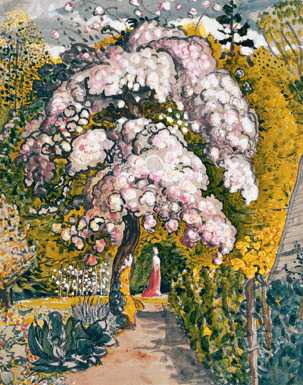This detailed description combines key elements from each person's voice captions:

This is a small oil painting, approximately two inches wide and three inches high, depicting a young maiden standing under an arch-like tree in a forest. The central focus is a tree with white and pink, cotton candy-like blossoms, symbolizing a flowering fruit tree. The tree has a curved brown trunk with touches of yellow. Above, the sky is overcast with various shades of gray clouds. A winding path, grayish-brown in color, leads from the foreground to where the maiden stands. The maiden wears a dress that is dark pink at the bottom, transitioning to white at the top, possibly indicating a white shirt. She stands at the end of the path, slightly to the right of the arch formed by the main tree. Along the path are green shrubs and plants in different shades of green, along with other trees bearing yellow and green foliage in the background. The painting skillfully captures the serene, wooded area under dim, overcast light.